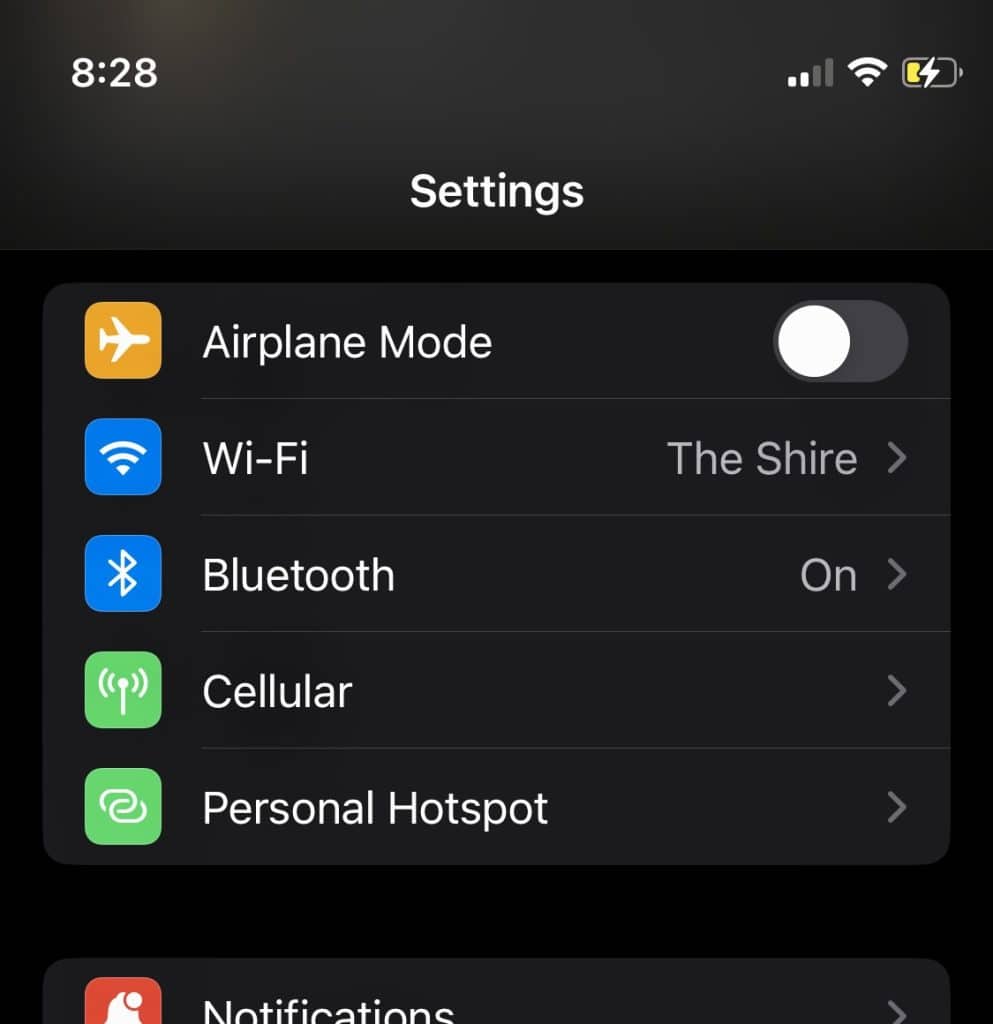This is a detailed screenshot from either a phone or a tablet's settings menu. At the top of the screen, there is a dark gray strip displaying the time '8:28' in white text. To the far right of this strip, there are several icons indicating connectivity and battery status: two out of four bars for the cellular network, a full Wi-Fi signal, and a battery icon showing approximately one-third charge remaining.

Below this top strip, centered in white text, the word "Settings" is displayed against a slightly darker background.

The main section of the screen showcases a list of settings, each within a distinct rectangular box with rounded edges against a black background:
1. **Aeroplane Mode**: A dark yellow square icon with a white airplane is on the far left, labeled "Aeroplane mode" next to it. The toggle switch for this feature is currently set to the off position (left).
2. **Wi-Fi**: A blue square icon with a white Wi-Fi signal symbol is displayed. Next to it, labeled "Wi-Fi", it amusingly indicates that the Wi-Fi network is named "The Shire".
3. **Bluetooth**: A blue square icon with the white Bluetooth symbol. The adjacent text reads 'Bluetooth' and indicates that Bluetooth is turned on.
4. **Cellular**: An icon of signal bars is displayed, alongside the label "Cellular".
5. **Personal Hotspot**: A green square icon with a white link chain depicts the "Personal Hotspot" setting.
6. **Notifications**: A red square icon with a white bell symbol appears, accompanied by the label "Notifications".

This meticulous caption ensures each element of the screenshot is described, providing a clear and comprehensive understanding of the visuals.